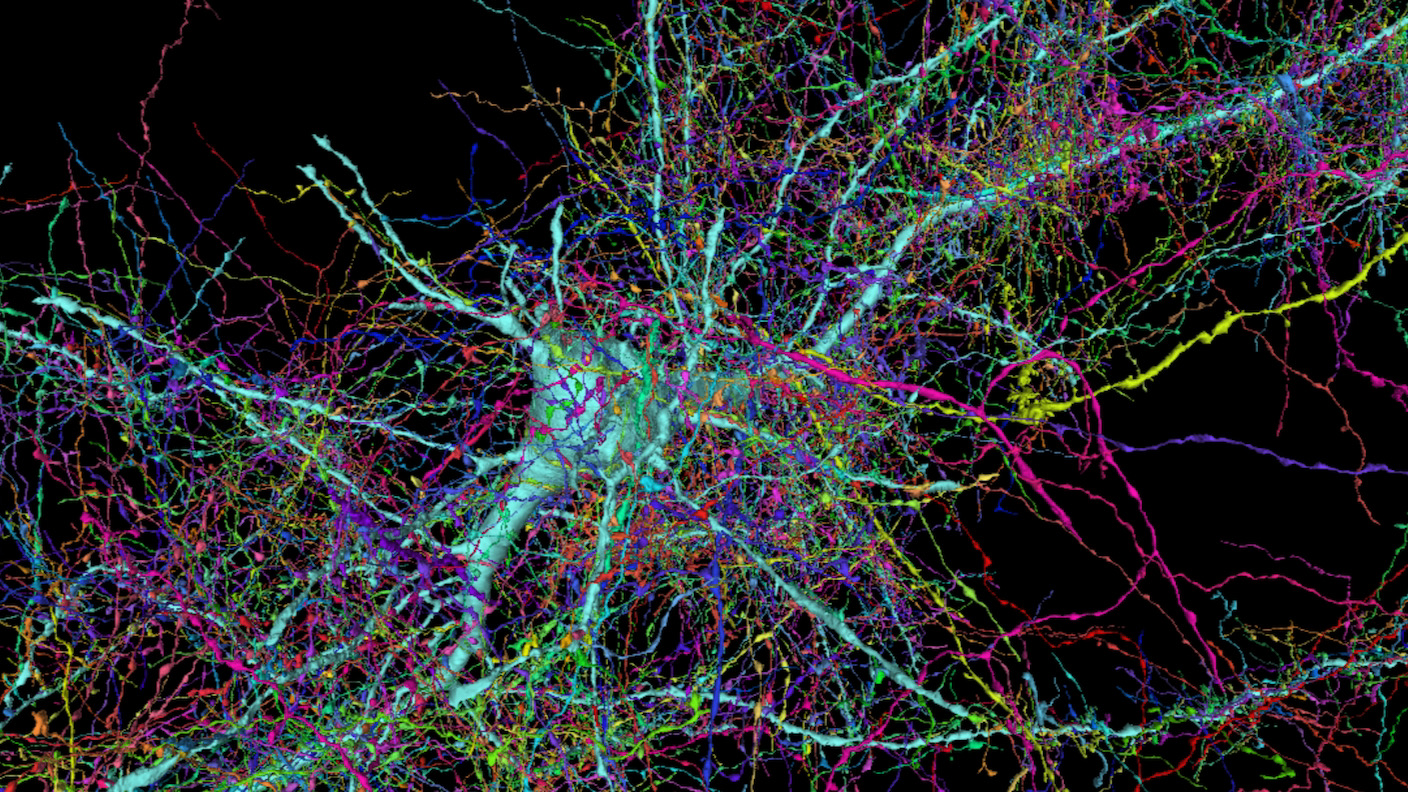This is an image on a black background, resembling a complex and vibrant neural network or tree roots. The image is rectangular, approximately six inches wide by three inches high. It features dense, multicolored striations and streaks converging into a central mass, which appears as the origin or "root" of the network. This central area is prominently blue, with large, thicker branches radiating in all directions, most notably extending towards the lower left and upper right corners of the image. Surrounding this core are numerous strands in shades of purple, pink, yellow, and three different greens, creating a mesmerizing tapestry of colors. The dense network of lines covers most of the black background, though areas in the upper left and lower right corners remain largely untouched, providing stark contrast. This visual display, reminiscent of an electrified nebula or an intricate web of brain waves, showcases the dynamic interplay of color and form.